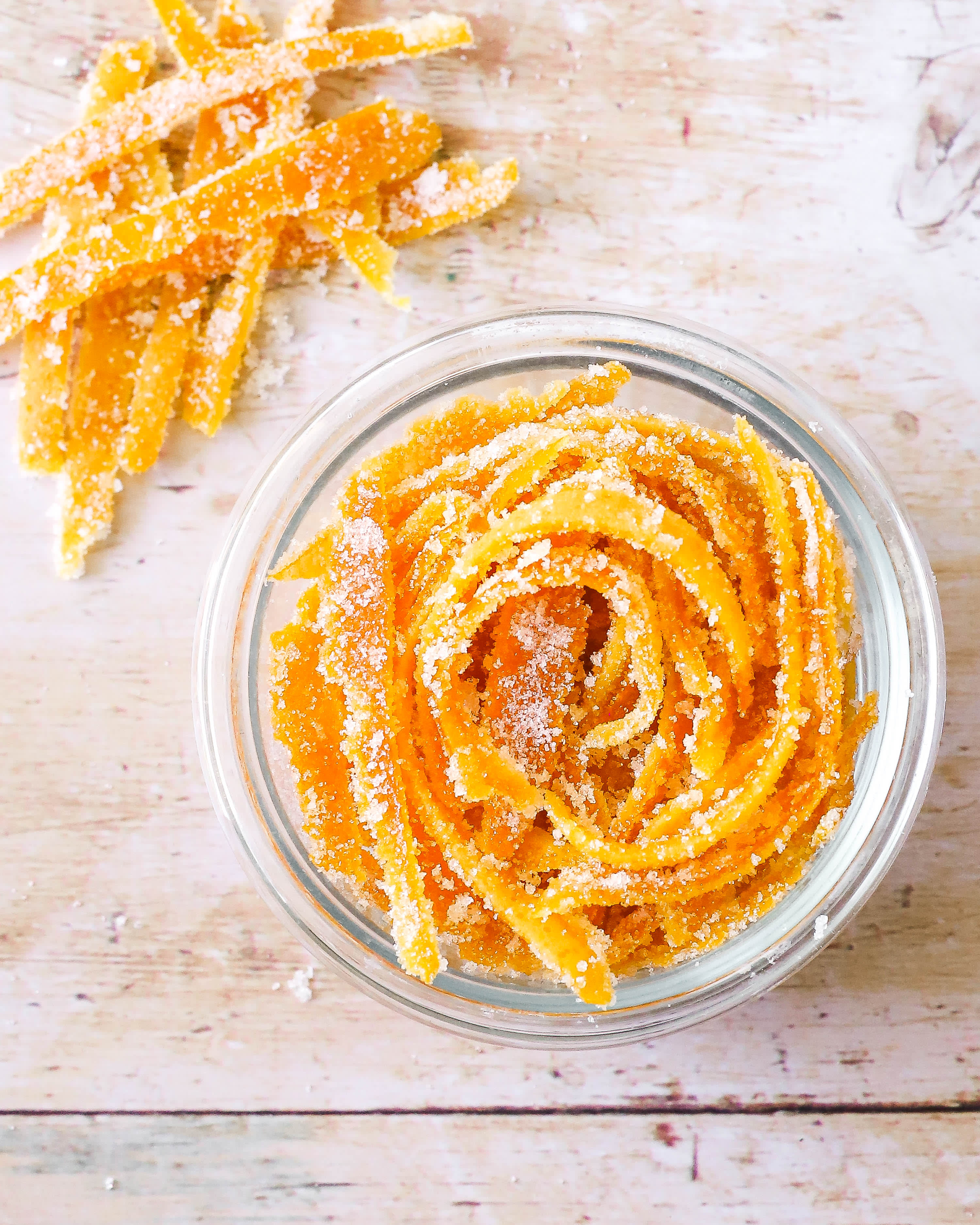The image showcases a small, clear glass dish filled with a spiral arrangement of bright orange, candied orange peels, coated generously in glistening white sugar reminiscent of snow. The dish, occupying the majority of the center of the frame, sits on a whitewashed, rustic wooden table that exudes a cozy, farmhouse charm. To the top left of the dish, several strips of candied orange peels are scattered haphazardly, enhancing the inviting and homemade aesthetic of the scene. The vivid orange hue and the sugary coating make the peels appear luscious and almost fragrant, as if you could smell their citrusy aroma wafting through the air. The overall brightness and simplicity of the composition draw attention to the delicate texture and vibrant color of the candied peels, highlighting their artisanal and delightful appeal.